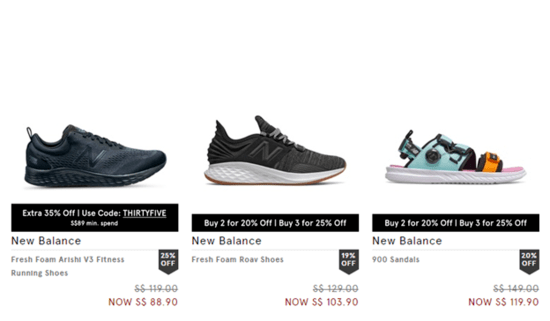**Screenshot from a New Balance Shoes Website**

*Image Description:*

The screenshot showcases three different listings for New Balance shoes.

1. **Black Sneaker:**
   - **Appearance:**
     - The sneaker is completely black.
   - **Promotions:**
     - There is a black rectangle below the sneaker with the text: "Extra 35% off, use code 35." Further text underneath suggests "min spend," but is difficult to read.
   - **Details:**
     - Background: White
     - Model Name: "New Balance Fresh Foam Arishi v3 Fitness Running Shoes"
     - Additional Offer: "25% off" displayed on a tab to the right.
   - **Pricing:**
     - Original Price: $119 (crossed out in gray)
     - Discounted Price: $88.90 (shown in red)

2. **Black and White Shoe:**
   - **Appearance:**
     - The shoe features a black upper half and a white bottom half.
   - **Promotions:**
     - A black banner reads: "Buy two for 20% off, buy three for 25% off."
   - **Details:**
     - Background: White
     - Model Name: "New Balance Fresh Foam Shoes"
     - Additional Offer: "19% off"
   - **Pricing:**
     - Original Price: $129 (crossed out in gray)
     - Discounted Price: $103.90 (shown in red)

3. **Colorful Sandal:**
   - **Appearance:**
     - The sandal features a teal main strap and back, an orange toe strap, a pink insole, and a white sole.
   - **Promotions:**
     - A black banner reads: "Buy two for 20% off, buy three for 25% off."
   - **Details:**
     - Model Name: "New Balance 900 Sandals"
     - Additional Offer: "20% off"
   - **Pricing:**
     - Original Price: $149 (crossed out in gray)
     - Discounted Price: $119.90 (shown in red)

Each listing includes promotional banners offering various discounts depending on the quantity purchased or specific promo codes.